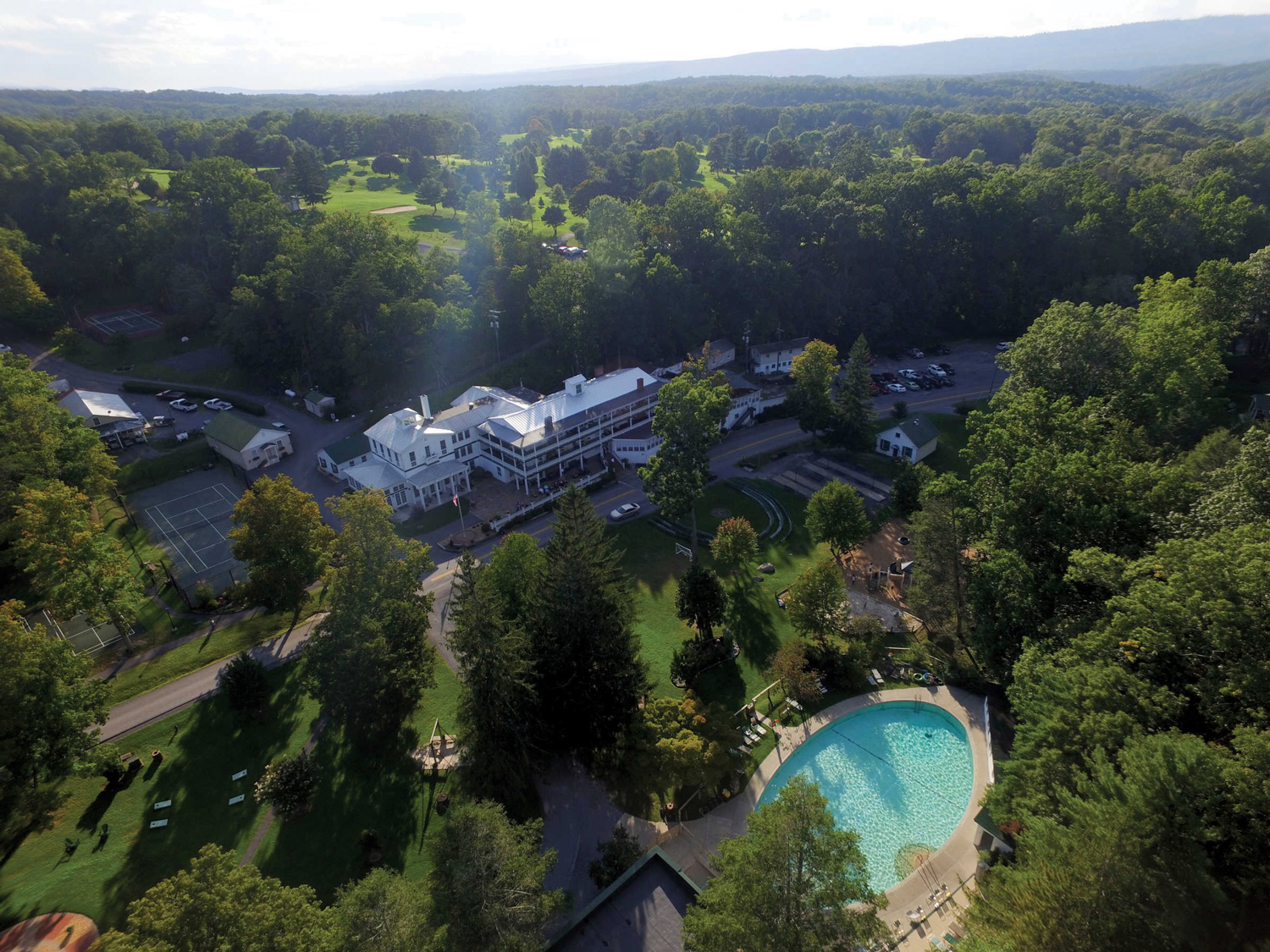This aerial or drone shot captures a sprawling, densely green town or city during the daytime. Sunlight filters through the clear white sky, casting patterns of light and shadow across the landscape. In the backdrop, a prominent hill ridge frames the horizon. The scene is populated with numerous white buildings, characterized by triangular roofs, and some with green rooftops. The multifaceted urban setting includes an interconnected villa or resort-like structure, featuring multiple floors with extensive balconies overlooking the area. 

Dotted amid the lush greenery are various recreational facilities: an oval-shaped swimming pool with vibrant light blue water sits in the foreground, surrounded by manicured lawns, tall trees, and dense foliage. Nearby, a double tennis court with a green surface is visible. A long blacktop road weaves through the greenery, where cars are intermittently passing. Further adding to the charm is a park area complete with people, benches, and well-maintained pathways. Towards the distant background lies a well-defined golf course, contrasting with the dense trees that permeate the area. The entire scene beautifully blends natural and urban elements, presenting a harmonized coexistence of greenery and structured development.